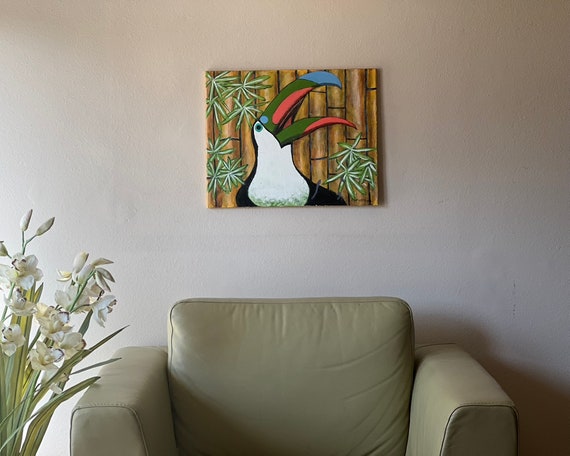This photograph captures a cozy, possibly indoor living space, likely a living room or waiting area, centered around a plush, low-set leather chair. The chair, light olive or beige in color with some wear and large armrests, is positioned directly beneath a captivating painting of a toucan. The chair is flanked on the left by a decorative arrangement of long-stemmed green plants and white flowers, partially illuminated by natural light, hinting at a nearby window outside the frame.

The toucan, the focal point of the artwork, is depicted with a striking color palette. It has a green beak adorned with red streaks and a blue tip, a characteristic white neck, and black feathers covering its body. The bird is set against a bamboo-themed background with green leaves, enhancing the tropical vibe of the scene. The toucan's head is tilted backward with its mouth wide open, adding a dynamic element to the painting, which hangs on a wall of light-colored paint, possibly beige or off-white. The room exudes a tranquil ambiance with its neutral tones and the vibrant, colorful accent provided by the toucan painting, making it a visually appealing and serene corner.